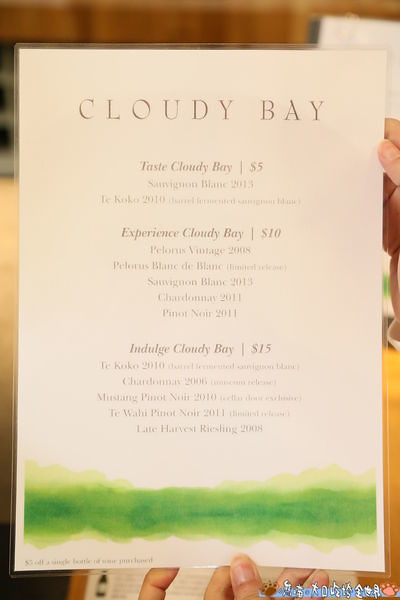In this photograph, a person's hand is seen holding a rectangular beige cardstock drink menu. The top of the menu is titled "Cloudy Bay," and following this, it lists various experiences with associated prices: "Taste Cloudy Bay" for $5, "Experience Cloudy Bay" for $10, and "Indulge Cloudy Bay" for $15. Each category features a variety of different wines and drinks. The bottom of the menu is adorned with a green watercolor brushstroke, resembling grass, adding an artistic touch to the overall design.